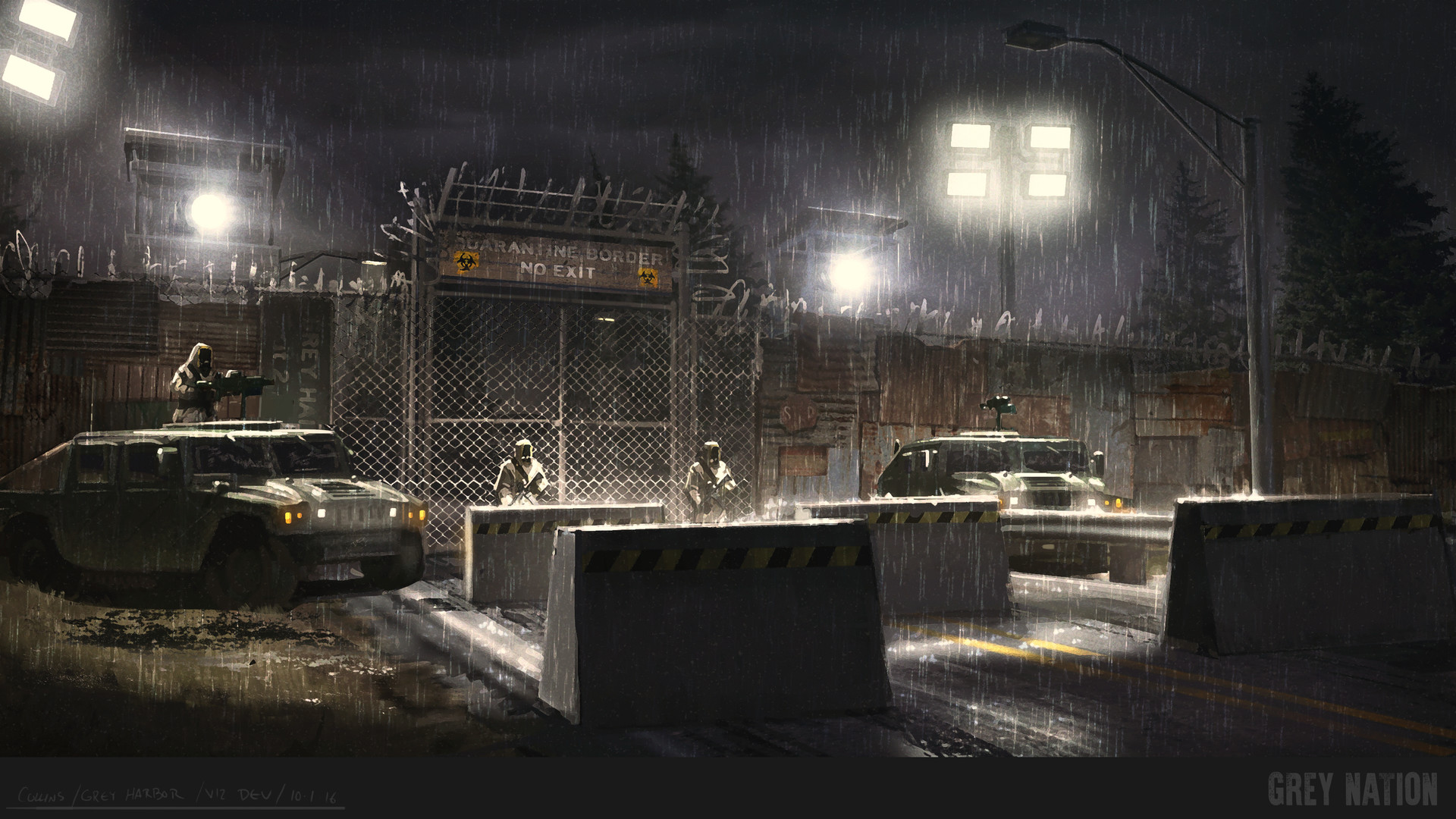In this digital rendering designed for a video game, a heavily secured military base or quarantine border is depicted in the midst of a heavy nighttime downpour. The rain falls straight down, indicating little to no wind. The base is fortified by large, rusted metal walls that appear haphazardly assembled and topped with barbed wire. Standing guard are three figures dressed in hazmat suits, each wielding guns, with spotlights and floodlights illuminating the area. Two military vehicles resembling Humvees are present, one with a soldier manning a gun turret. The scene is further secured by four large concrete barricades placed across the road leading up to the gate. A makeshift sign reading "Quarantine Border No Exit" with radiation symbols is prominently displayed. The image is characterized by a dark, gloomy aesthetic with the phrase "Gray Nation" written in gray text on a dark gray bar in the lower right corner. Additional, but illegible, handwritten text resides in the lower left.